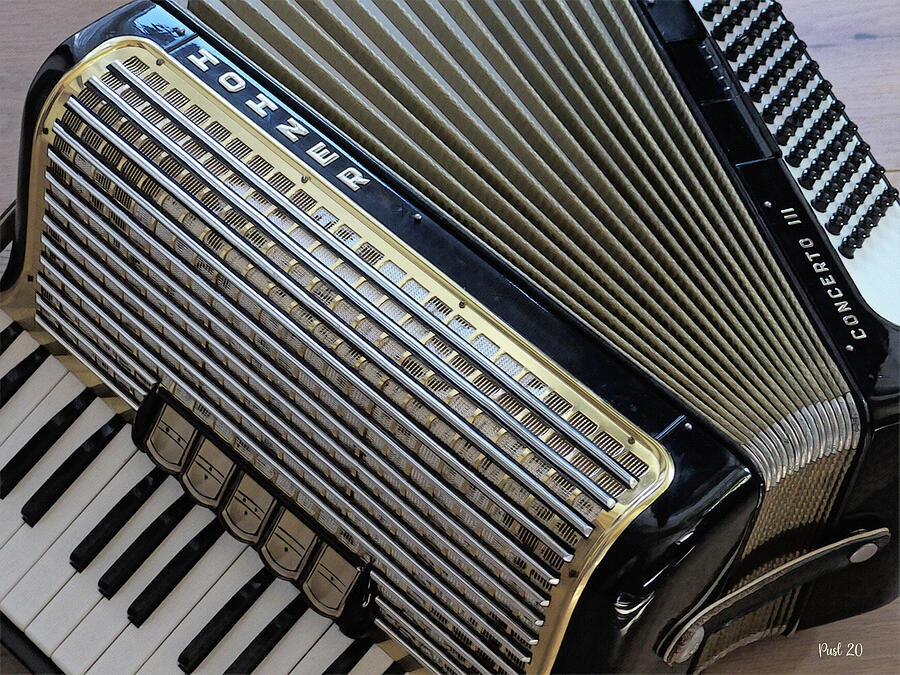This detailed close-up image captures a Hohner accordion with a black, shiny finish and gold accents. The centrally placed keyboard features white and black keys, partially cut off at the top and bottom edges of the photo. Above the keyboard, a gold-colored or brass-toned speaker grille with silver metallic bars allows sound to emanate from the instrument. The accordion's bellows, resembling a paper fan, are slightly compressed in this shot and bear the label "Concerto III" on the lower movable part. The top portion of the image reveals rows of black buttons on a white base, used to control different keys and tones. Along the side of the accordion, the brand name "Hohner" is prominently displayed in gold letters. In the bottom right corner, the image is overlaid with white text reading "Fine Art America" followed by "Pushes 20," though parts of it are too small to be clearly deciphered.